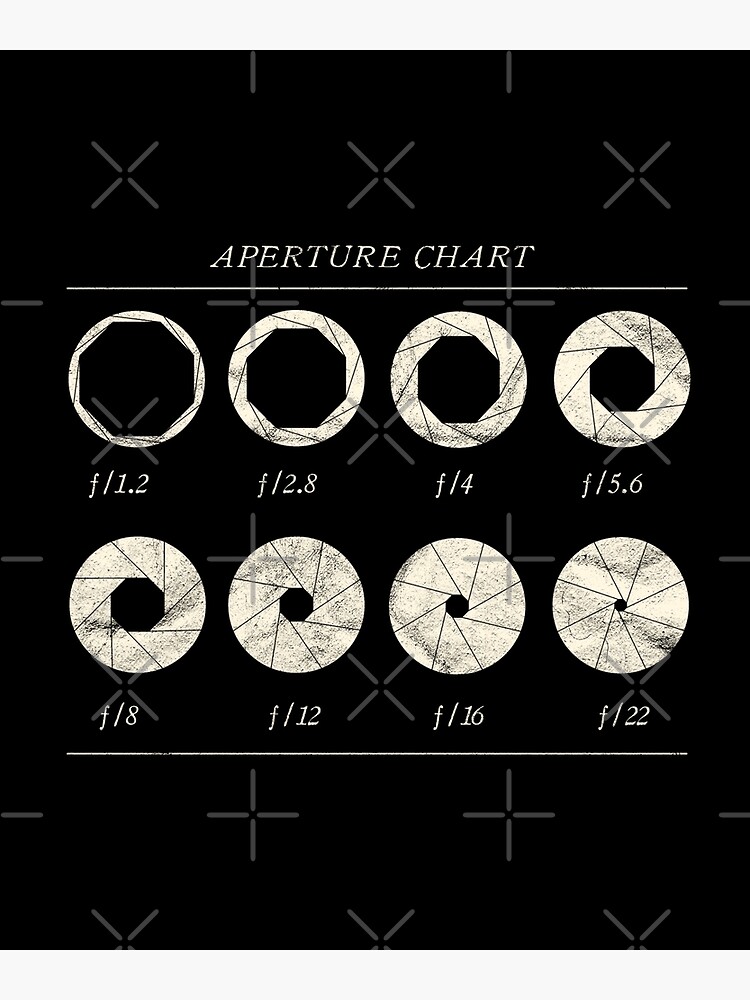The image displays an "Aperture Chart" on a black background adorned with light gray X and plus sign graphics, creating a subtle, textured watermark effect. Centered in the image are eight hexagon-like shapes enclosed in circles, each with varying levels of shading, symbolizing different aperture sizes. The silhouettes represent apertures labeled as F/1.2, F/2.8, F/4, F/5.6, F/8, F/12, F/16, and F/22 in white text. There is a solid white line above and below these aperture symbols, and the chart title "Aperture Chart" is prominently displayed at the top in white capital letters. The overall design is structured and schematic, mimicking the appearance of a camera shutter.